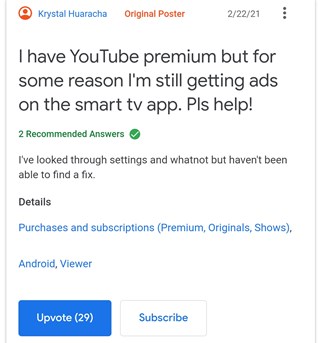A screenshot from an online forum where users can ask questions and receive answers from the community. At the top left corner, the profile of the original poster, Crystal Huaracha, is displayed. The post, made on February 22, 2021, poses the question: "I have YouTube Premium but for some reason, I'm still getting ads on the Smart TV app. Please help."

Beneath the question, in green text, it states "2 recommended answers." Following this, Crystal provides additional context: "I've looked through settings and whatnot, but haven't been able to fix it."

The category, labeled in blue as "Details," clarifies that the question relates to "Purchases and subscriptions (Premium, Original Shows)" as well as "Android viewer." At the bottom, there are two buttons – a blue "Upvote" button showing "29" votes, and a "Subscribe" button.